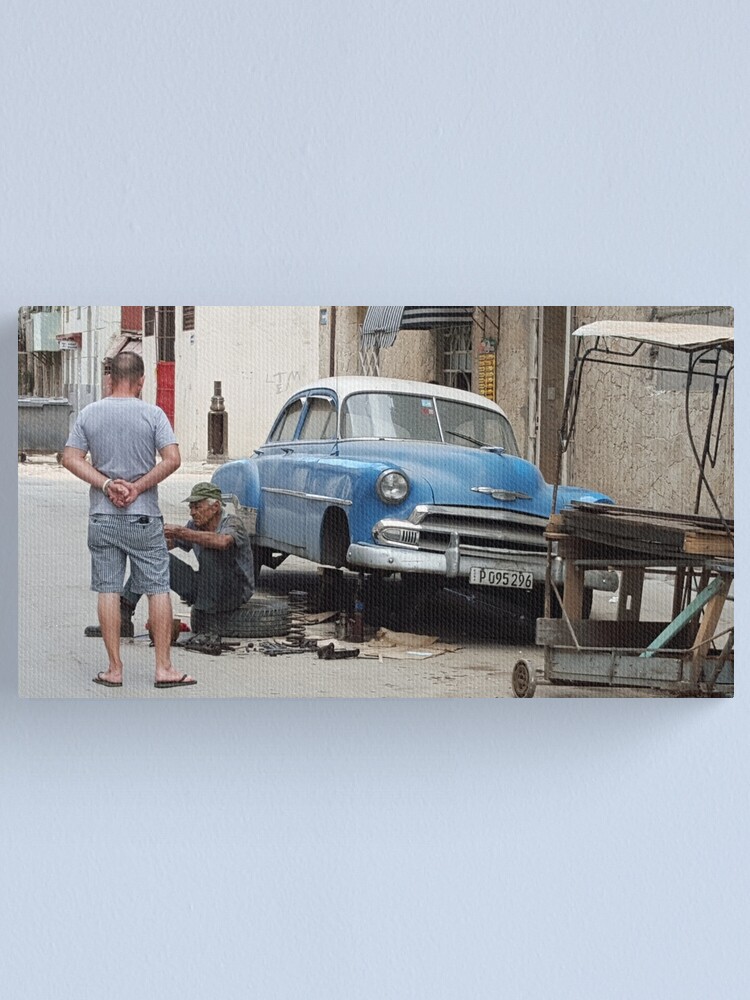In this photograph, a detailed scene unfolds in a foreign alley, featuring two men working on a classic 1950’s blue car with white accents and a chrome grill. The car, possibly a Chevy, is jacked up with its tire removed, tools and tires scattered around. The older man, presumably the owner and mechanic, sits on a tire wearing black pants, a gray t-shirt, and a green cap, his white hair contrasting against the alleyway's backdrop. His companion, a younger, almost bald man dressed in gray shorts, a gray t-shirt, and flip-flops, stands nearby observing the repair process. The front license plate reads "P095296" and hints at an international setting, possibly Cuba. In front of the vehicle, a piece of unidentified equipment or buggy adds to the bustling atmosphere of this rustic locale.